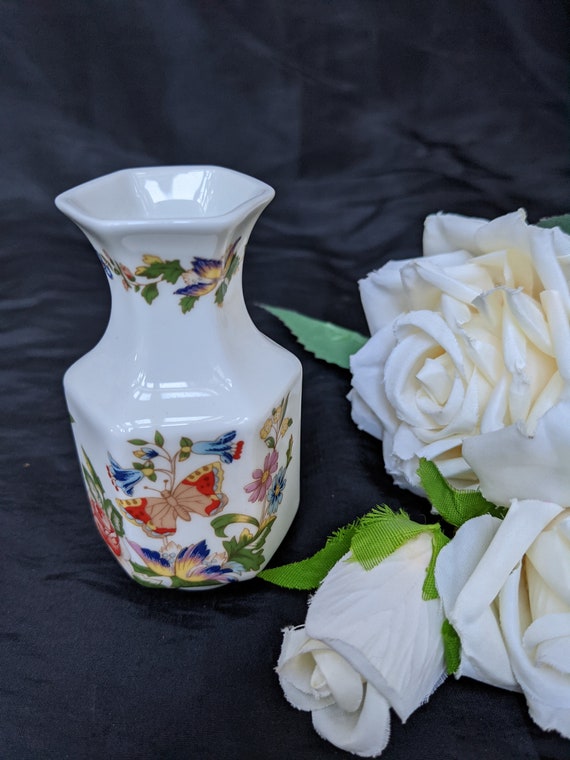The image presents a pristine white ceramic vase, characterized by its shiny, glossy finish that catches the light beautifully. Adorned with intricate patterns featuring a vibrant array of butterflies and flowers, the vase showcases a butterfly with coral and red wings accented by hints of yellow, alongside an assortment of multicolored flowers in pink, blue, yellow, and purple hues. Green leaves add a natural pop of color to the design. The vase rests on a dark, potentially purple, blanket or carpet, set against a backdrop of a black curtain. Accompanying the vase are artificial white flowers, including a large and a smaller fabric rose, with green leaves, arranged next to it as part of the display. The vivid and diverse colors on the vase contrast the dark background, highlighting its detailed artwork and making the setup visually appealing.